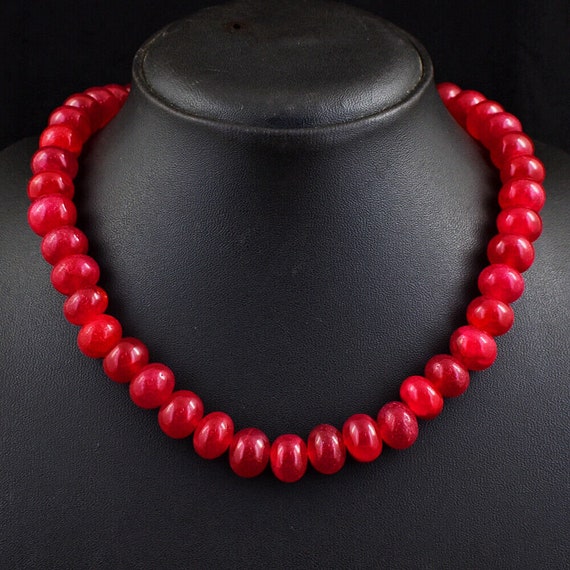The image depicts a close-up of a red beaded necklace draped around a black mannequin bust. The background is also black, but due to strategic lighting, white highlights accentuate the neck area of the mannequin. The mannequin has no head, focusing instead on the neck and upper chest, revealing intricate leather stitching where the neck is cut off. The necklace consists of red, oval-shaped beads that vary slightly in size and shade, ranging from a deep red to reddish-pink, with some beads reflecting light, creating a subtle glare. The beads are evenly spaced and connected, forming a continuous loop around the neck of the mannequin.